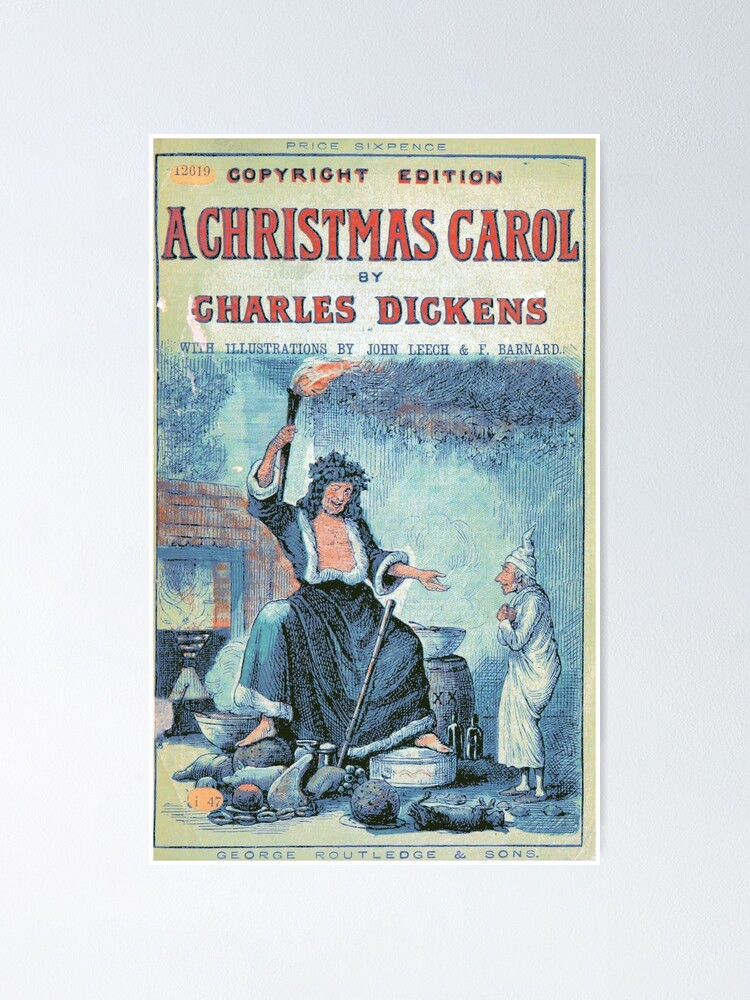This image depicts a framed, possibly expensive piece of artwork showcasing the cover of the copyright edition of "A Christmas Carol" by Charles Dickens. The top part of the cover in small letters includes "Price: Six Pence" and "12619." The main title, "A Christmas Carol," is prominently displayed in large, red capital letters, followed by "by Charles Dickens." Below that, it states in smaller print, "with illustrations by John Leach and F. Barnard." The illustration on the cover features a large, ghostly man holding a flaming torch in his right hand, extending his left hand towards a smaller man, who appears to be pleading with him. The scene gives an impression of another era, with white dishes scattered around the background and stones in front of the characters. The smaller figure, likely in nightclothes, represents Charles Dickens, gazing at the ghost. The bottom of the cover mentions "George Routledge and Sons" in small letters. Overall, the image presents an evocative, detailed portrayal aligned with the classic, timeless feel of the story.